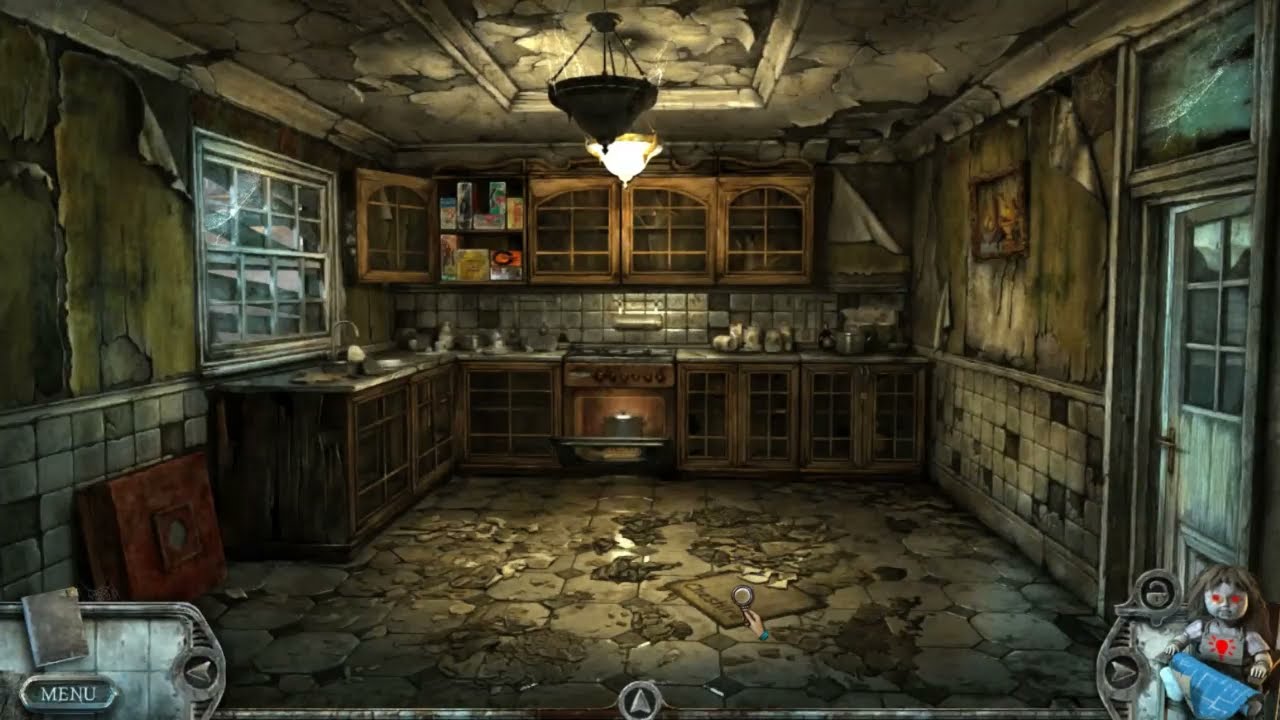The image appears to be a screenshot from a horror-themed video game, depicting a completely rundown kitchen that looks abandoned and neglected. The kitchen is in a state of severe disrepair: the floor is rough and dirty, likely made of worn-out stone, and the ceiling is torn apart with remnants of white wallpaper barely holding on, from which a single light fixture dangles and is still lit. The background features brown-edged cabinets with empty glass panes and decorative brown lines, all of which are empty. Torn greenish wallpaper clings to the walls, adding to the deteriorated atmosphere. In the bottom left-hand corner of the image, "MENU" is displayed inside a silver square. On the right-hand side, there is a creepy-looking doll with red eyes and gray hair, contributing to the eerie setting. The overall color scheme of the image includes shades of black, white, gray, blue, red, and yellow. The chaotic disarray, coupled with the unsettling doll, strongly suggests that the game is set in a horror context.